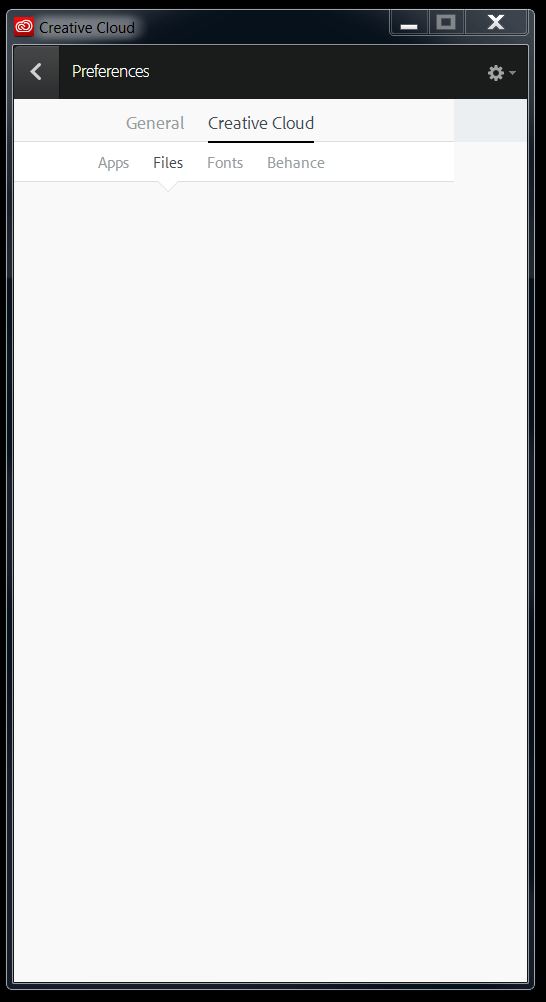The image displays the interface of Adobe Creative Cloud on a mobile device, likely a smartphone or tablet. The background is predominantly black, forming a large rectangular area around the central white content box. The black border is thicker at the top and thins out to a narrow strip around the sides and bottom of the white rectangle. 

At the top of the black border, the text “Creative Cloud” is visible, along with the Creative Cloud logo, which features two stylized letter C's back-to-back in red, forming a cloud shape. Adjacent to this, you can see the window control icons: a minimization button, a full-screen button, and an X (close button).

Within the white content area, on the upper left, there's a left-pointing arrow icon. Moving to the right, you'll find the word "Preferences" inside a black box with white text. Further to the right is a gear icon that opens a dropdown menu. 

Below this top section, the interface displays a series of tabs: "General," "Creative Cloud," "Apps," "Files," "Fonts," and "Behance." This capture meticulously illustrates the navigational and functional structure of the Adobe Creative Cloud application on a handheld device.